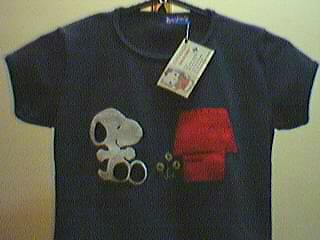Displayed against a tan-colored wall, this image features a children's dark navy t-shirt as its focal point. The backdrop exhibits subtle variations in shading, with the lower left corner appearing slightly darker due to the shadow cast by the shirt, influenced by the lighting in the scene. The t-shirt itself is designed with quarter-length sleeves and features a charming illustration of Snoopy standing next to his iconic red doghouse. Adjacent to the doghouse are three small yellow flowers, adding a touch of color to the design. Snoopy is depicted in his classic white body with black ears and feet. The red doghouse is distinguished by its rectangular shape and parallelogram-patterned roof. A white tag hangs from the neck of the shirt, adorned with an image of Hello Kitty, although the accompanying text is not legible.